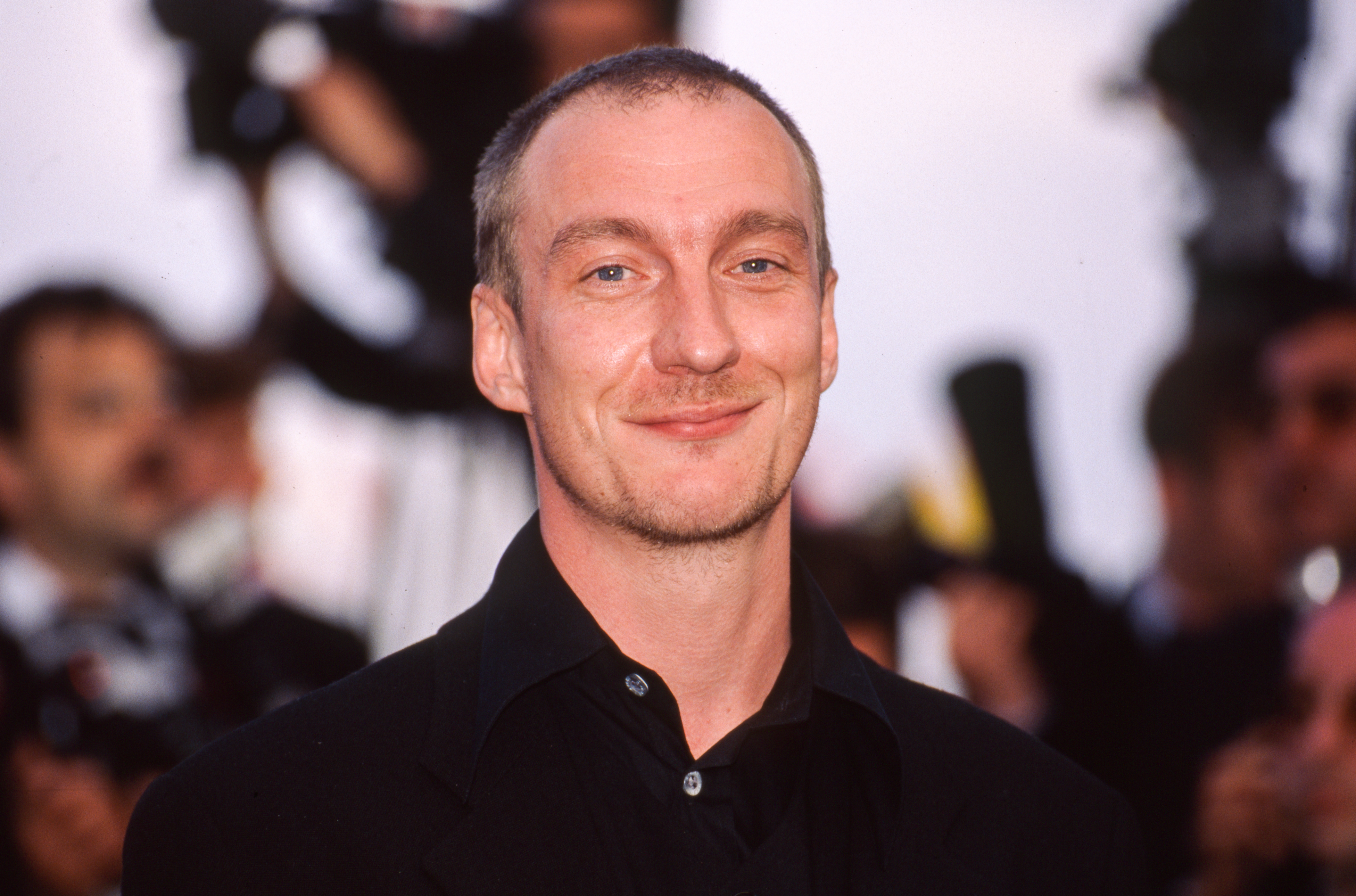The image captures an outdoor event, possibly a press gathering, movie premiere, or award show, marked by a blurred background filled with indistinguishable figures dressed predominantly in black and white. Central to the image is a smiling man with blue eyes, recognized as an actor, who sports short, thinning hair styled in a buzz cut. His facial hair is a light mustache and a subtle five o'clock shadow extending to his neck. His attire consists of a black button-down shirt, unfastened at the collar, layered beneath a matching black blazer. The photograph captures him from head to mid-chest, as he directs a slight smirk towards the photographer, exuding a casual yet composed demeanor.